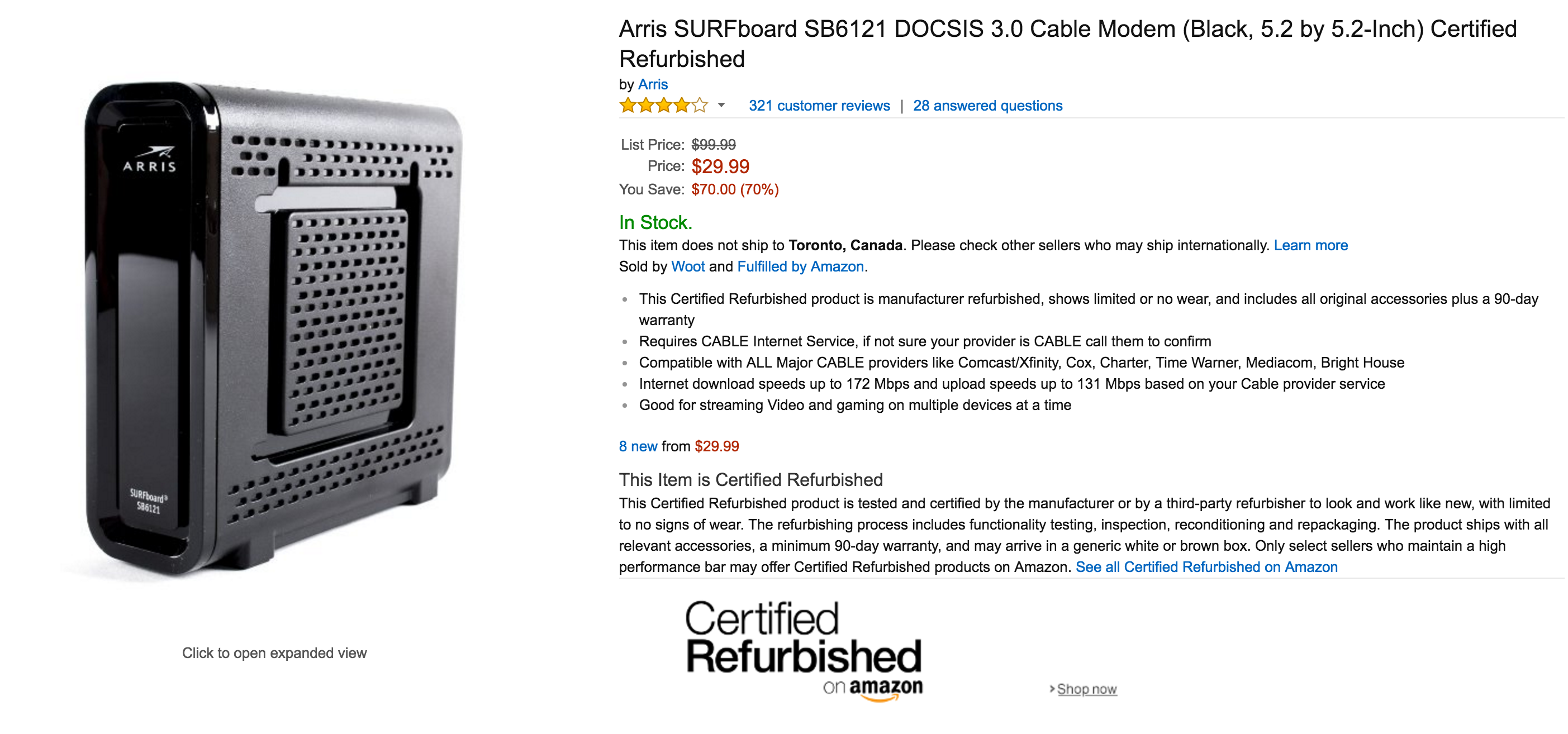The image is a screenshot of an Amazon product listing. At the top, it displays "Armus Surfboard" and includes specifications such as "3.0 Cable Modern Black," with dimensions "5.2 by 5.2 inches," and the label "Certified Refurbished." The product has a rating of 4 out of 5 stars, based on 321 customer reviews and 28 answered questions. A prominent feature is the large "Certified Refurbished on Amazon" text at the bottom. The listing indicates the price as $29.99, boasting a 70% discount, saving customers $70 off the original price. It confirms the item is in stock with green text. A note specifies that the item does not ship to Toronto, Canada, accompanied by a "learn more" link. Additionally, it mentions that there are eight new items available from $29.99. There is also a clickable link labeled "See all certified refurbished on Amazon." The image allows users to click to expand the view for a closer look at the product.